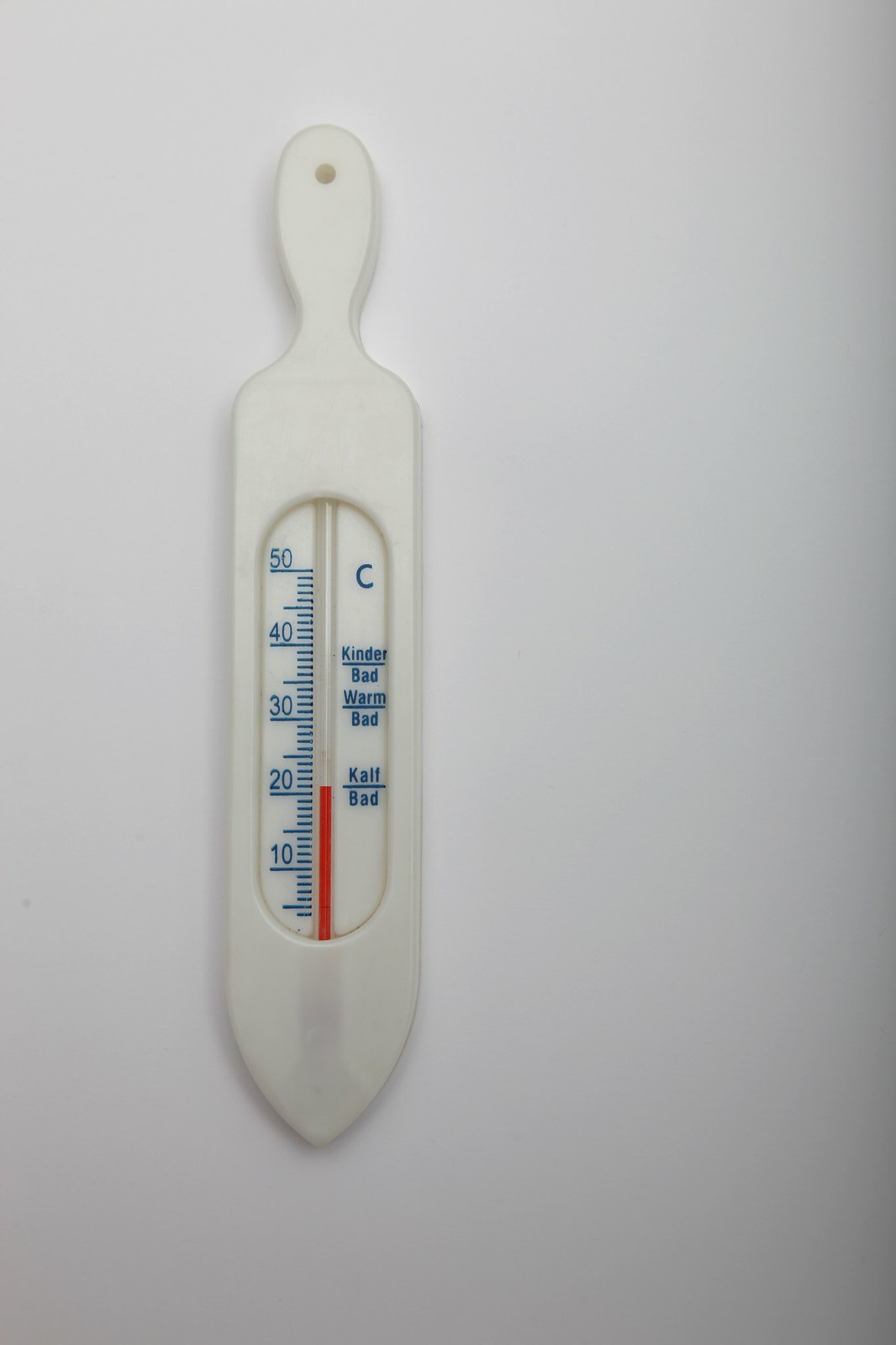This image features a white plastic thermometer designed in an unusual shape reminiscent of a cutting board. It includes a handle at the top with a hole, allowing it to be easily hung on a wall. The thermometer displays temperatures in Celsius, marked with blue numbers at intervals of 10, from 10°C to 50°C. A transparent strip runs down the center, containing a red mercury-style line that rises to indicate the temperature. 

The thermometer has various sections labeled in German: "KINDER BAD" (translated to 'Children's Bath'), "WARM BAD" ('Warm Bath'), and "KALF BAD" ('Cold Bath'), each corresponding to different temperature ranges. The background of the image is a clean, white surface, highlighting the thermometer against it. The overall setup and detailed labeling make it clear and easy to read, providing precise temperature measurements for different uses.